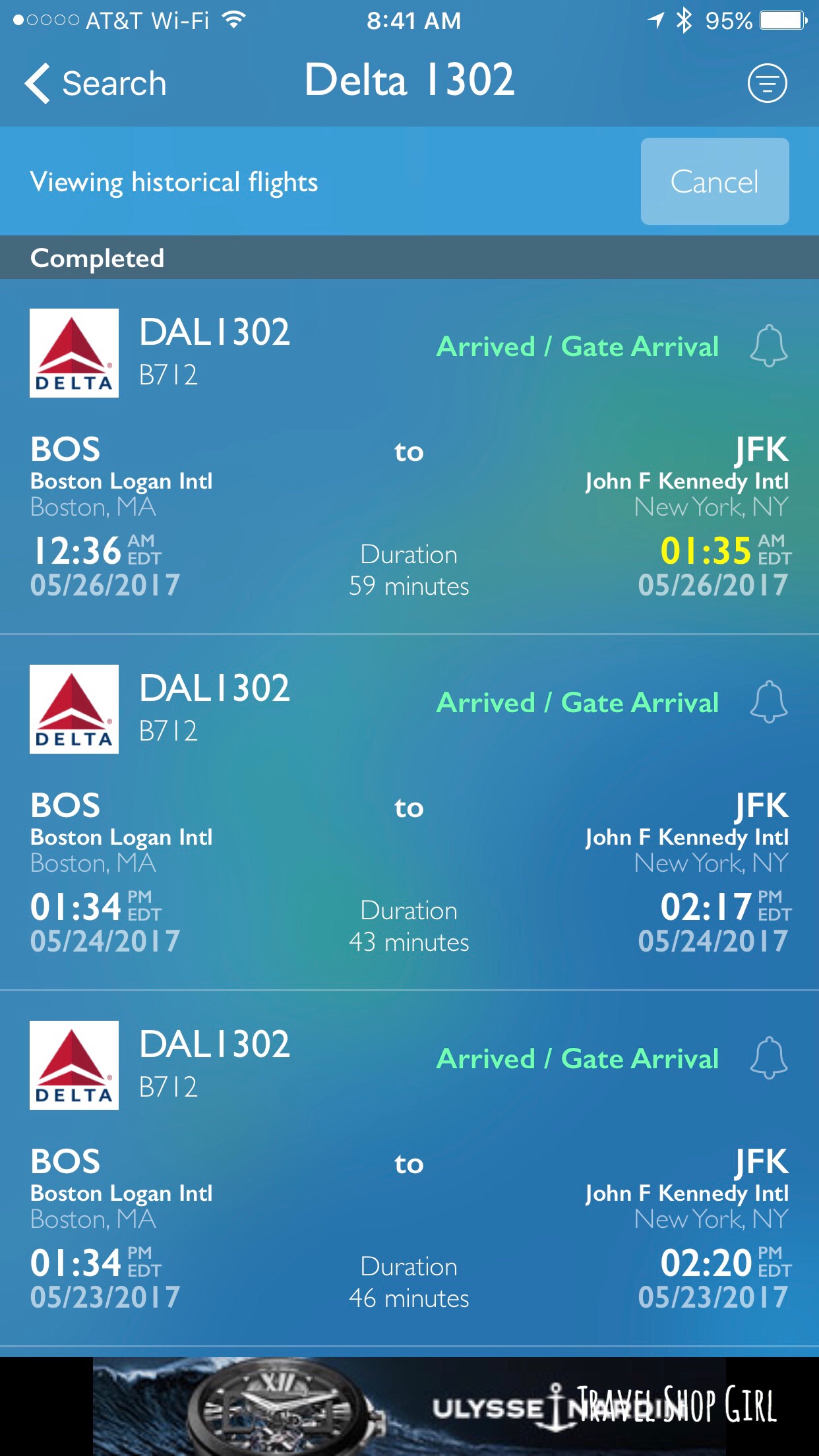**Mobile Screenshot of Delta Flight Information**

The mobile screenshot showcases detailed flight information against a completely blue background. At the top, there is a header that reads "Delta I-303," alongside a search option that indicates the ability to go back. The screenshot was taken at 8:41 a.m., with the phone battery showing 95% charge.

Below the header, a blue bar labeled "Viewing Historical Flights" appears, accompanied by a cancel button on the right. Underneath this, a section titled "Completed" lists all Delta flights, identifiable by the white boxes featuring the Delta logo.

1. **Flight DAL-1302-B712**
   - Status: Arrived / Gate Arrival (in green)
   - Route: From Boston Logan International Airport (BOS), Boston, Massachusetts
   - Departure: 12:36 a.m., May 26, 2017
   - Destination: John F. Kennedy International Airport (JFK), New York, New York
   - Arrival: 1:35 a.m. EDT, May 26, 2017
   - Duration: 59 minutes

2. **Flight DAL-1302-B712**
   - Route: From Boston Logan International Airport (BOS), Boston, Massachusetts
   - Departure: 1:34 a.m. EDT, May 24, 2017
   - Destination: John F. Kennedy International Airport (JFK), New York, New York
   - Arrival: 2:17 p.m. EDT, May 24, 2017
   - Duration: 43 minutes

3. **Flight DAL-1302-B712**
   - Status: Arrived / Gate Arrival
   - Route: From Boston Logan International Airport (BOS), Boston, Massachusetts
   - Departure: 1:34 p.m. EDT, May 23, 2017
   - Destination: John F. Kennedy International Airport (JFK), New York, New York
   - Arrival: 2:20 p.m. EDT, May 23, 2017
   - Duration: 46 minutes